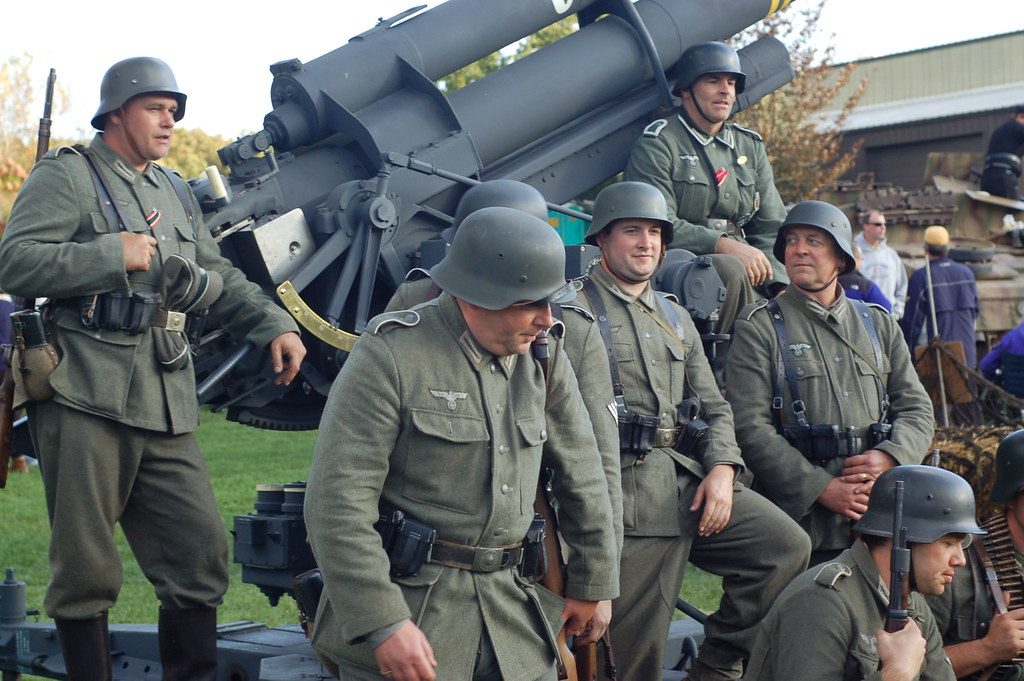A realistic, horizontally-oriented photograph taken outdoors during an overcast day features eight soldiers posing around a large black cannon aimed from the bottom left to the top right. The scene is set against a backdrop of yellow-leaved trees and green grass to the left, with a gray, warehouse-like building to the right. The soldiers, who appear to be white men in their 20s to 40s, wear World War I or World War II-style uniforms with plain green jackets, pants, and greenish-gray helmets. Some soldiers are holding rifles or have them slung over their shoulders, and a few are seen engaging in conversation while smiling. In the background, additional people dressed in modern clothing suggest this might be a reenactment or a historical event. The setting includes civilians observing the scene, adding an element of authenticity or historical portrayal to the photograph.